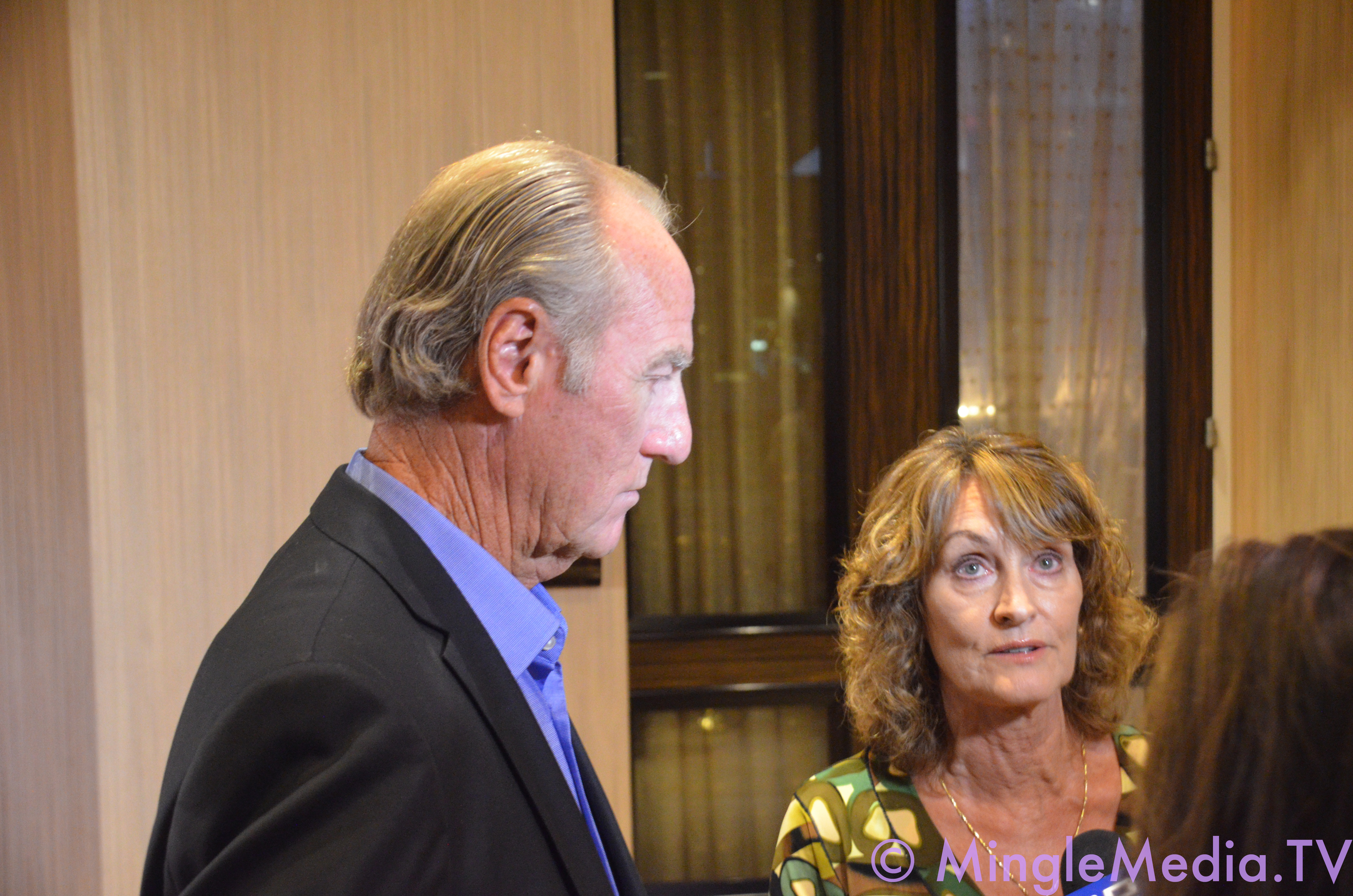In this image, we see an older actor on the left-hand side, recognized from both the 90s show "Coach" and his role as Dale on "Young Sheldon." He has gray, slicked-back hair that is thinning at the front. He is dressed in a black suit jacket over a blue button-down collared shirt. The background reveals a paneled wall with a window framed in wood and curtains on the opposite side. The bottom right of the image features a watermark with "copyright mingle media.tv." In front of the actor, there are two women. The first woman, with shoulder-length curly brown hair and bangs, is wearing a green and brown dress with a gold chain. The second woman, positioned slightly ahead, has dark brown hair.